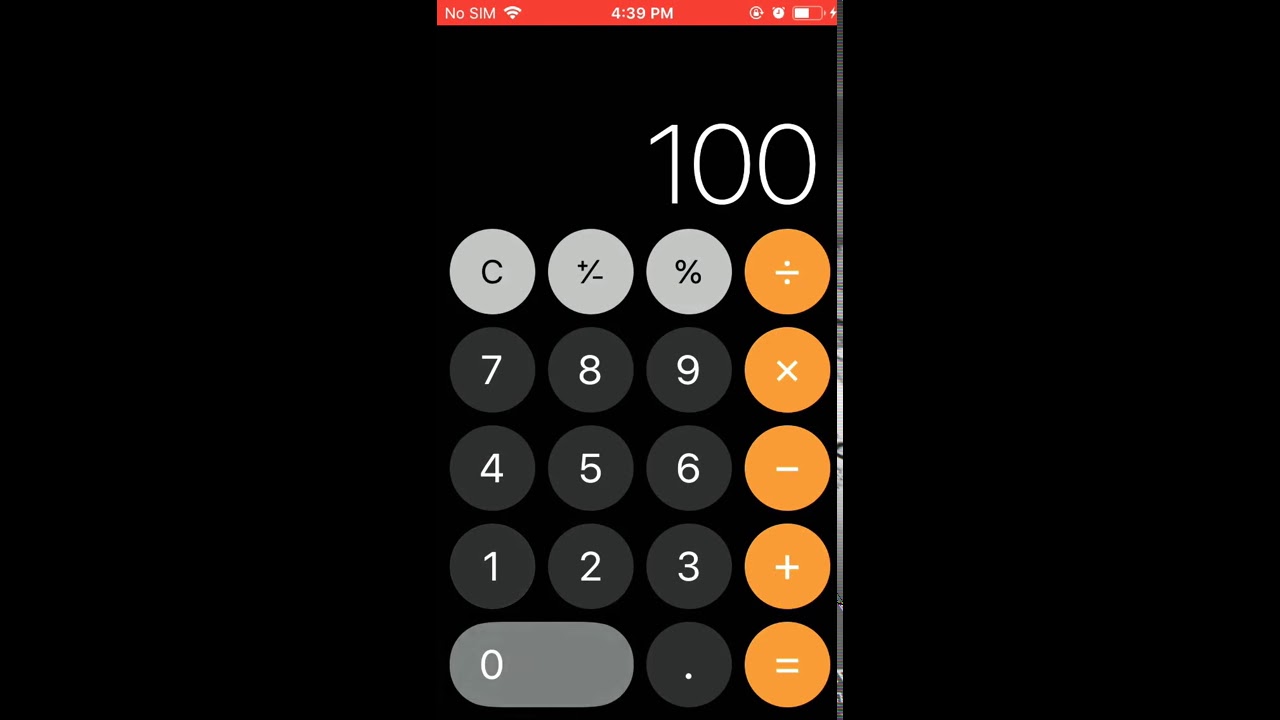A screenshot captures the calculator app on an iPhone operating in dark mode. The display shows the number "100 100," though the context of this entry—whether it was typed directly or results from a calculation—is unknown. The interface shown is the basic version, featuring a numerical keypad, a clear button, and options for positive/negative toggles, percentage, and basic arithmetic operations. Notably absent are any advanced scientific functions. 

In the notification area at the top of the phone screen, it reads "4:39 p.m." The battery icon indicates it is approximately halfway depleted. A red notification bar suggests a potential issue, such as no service or an emergency alert. Additionally, there is an alarm icon, indicating an active alarm setting.